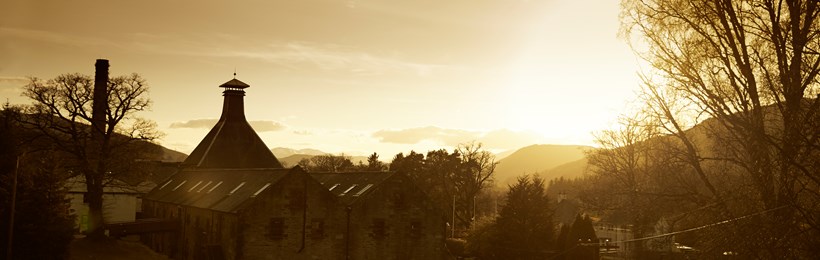At the golden hour of sunset, this photograph captures a serene landscape where the sun, positioned slightly right of center, casts a warm glow as it dips behind distant mountain peaks. On the far right, the graceful silhouette of an oak tree stands tall, its dark form contrasting against the colorful sky. To the left, the sharp steeple of a building pierces the twilight, descending into a two-story white structure with a dark roof adorned with skylights. A black post rises prominently to the left of these houses, contributing to the intricate foreground details. Amidst this scene, another oak tree stands behind the post, merging with the environment. On the right-hand side, additional trees create a natural frame for a multi-story white house nestled quietly in the background. The sky, adorned with a few wisps of fair-weather clouds, completes this picturesque tableau, embodying the tranquil beauty of sunset.